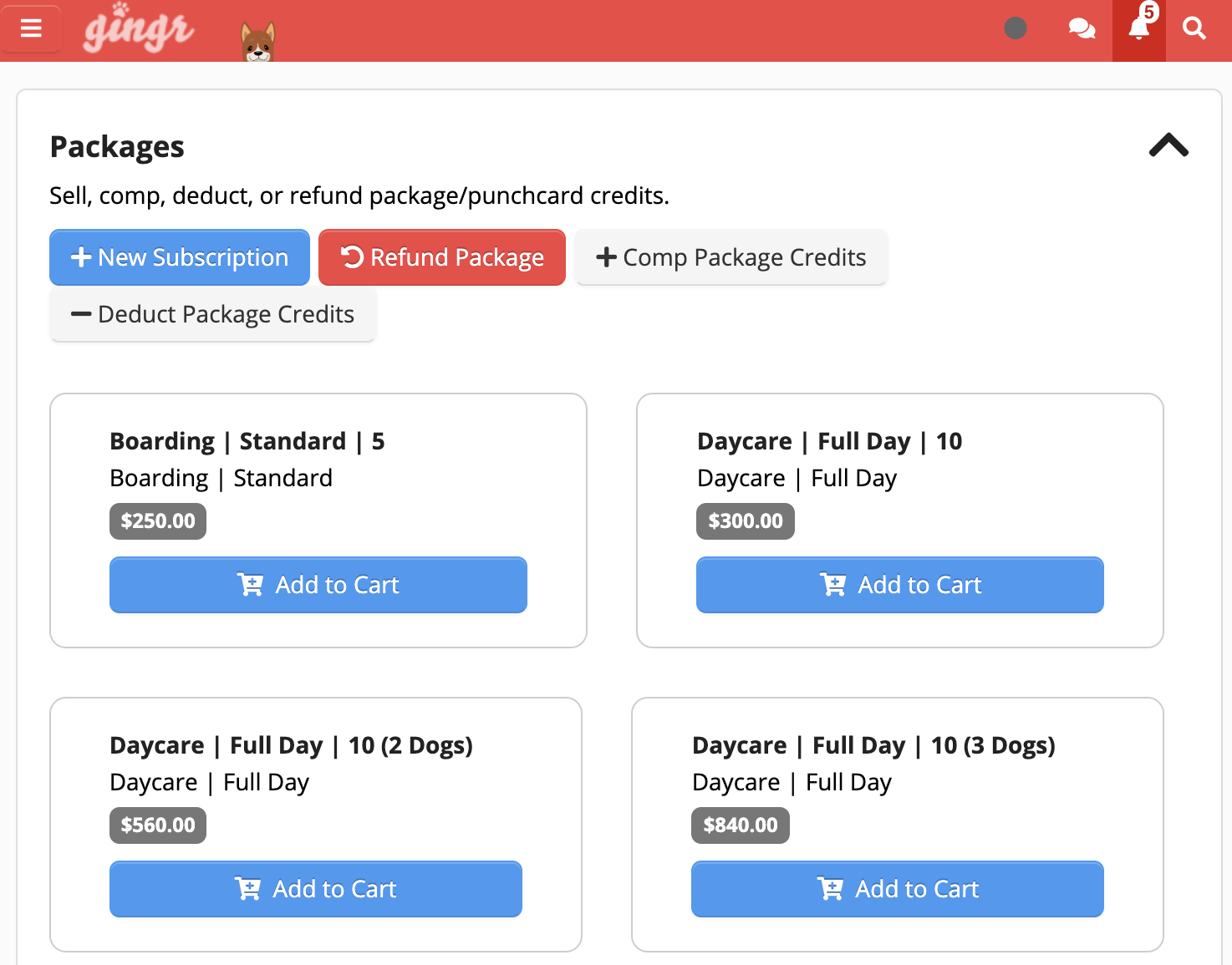This screenshot from a website features a product page layout. At the very top, there's a prominent horizontal red bar. To the left on this bar, a white menu button resides next to a white logo text that reads "Ginger" accompanied by a dog face icon. On the right side of this bar, there are three distinct icons: a chat button, a notification bell, and a search button.

Directly below the red bar, a white rectangular section spans horizontally. In the top left corner of this section, it lists categories such as "Packages" and options to "Sell, Comp, Deduct, or Refund Package/Credit Punch Cards." Beneath these headings, there are three buttons in different colors: blue, red, and gray, with an additional gray button situated below the blue button. These buttons correspond to functionalities for new subscription purchases or refunds, comp package credits, and deducting package credits. Further below, there are four "Add to Cart" buttons in varied color sequences: blue, red, blue, and blue again, ending with red.